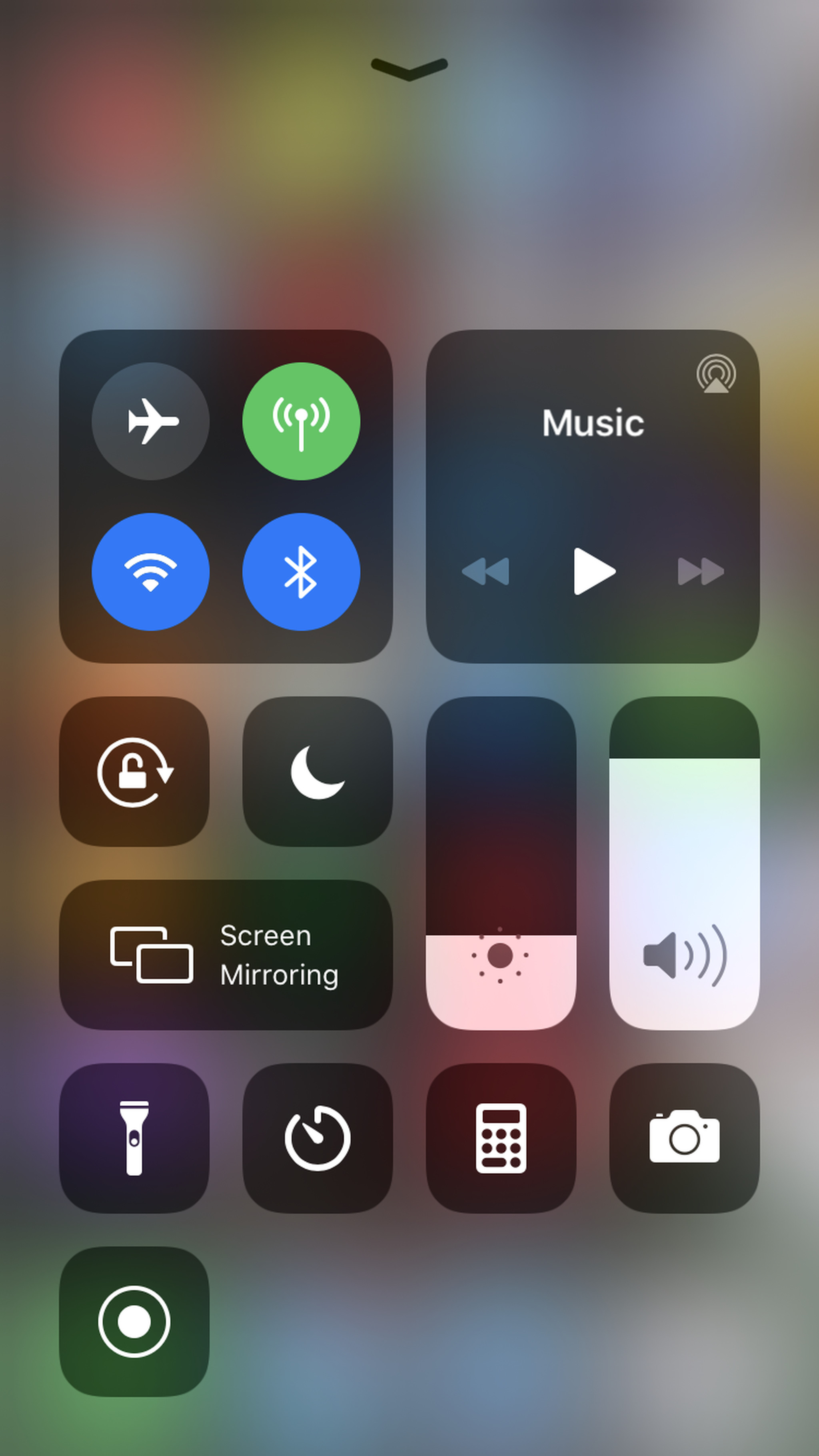The image depicts the icon of a smartphone interface against a blurred, grayish background accented with colored lights. The detailed breakdown of the interface elements is as follows:

1. **Upper Center:**
   - A downward-pointing arrow icon.

2. **Left Box:**
   - Comprises four icons arranged in a 2x2 grid.
   - **Top Row:**
     - Airplane mode icon.
     - Signal strength icon.
     - Green circular icon.
   - **Bottom Row:**
     - Blue circles depicting Wi-Fi and Bluetooth icons.

3. **Right Box:**
   - Features a signal icon in the upper right corner accompanied by the word "Music" in white text.
   - Contains three control buttons:
     - A white play button in the center.
     - Gray back and forward buttons flanking the play button.

4. **Lower Section:**
   - Multiple icon boxes are present, including:
     - A dark box with a moon (Do Not Disturb mode).
     - A locked padlock icon encircled by an arrow.
   - Two slider bars:
     - One for brightness adjustment marked with a sun icon.
     - One for volume control marked with a speaker icon.
   - An additional box for screen mirroring.

5. **Bottom Section:**
   - A row of icons for various utilities:
     - Flashlight.
     - Time.
     - Calculator.
     - Camera.
     - A circular icon that appears to be a target or focus symbol, depicted as a circle within a circle.

The overall interface layout is rich with functionality, indicated by the detailed icons and controls available for the user.